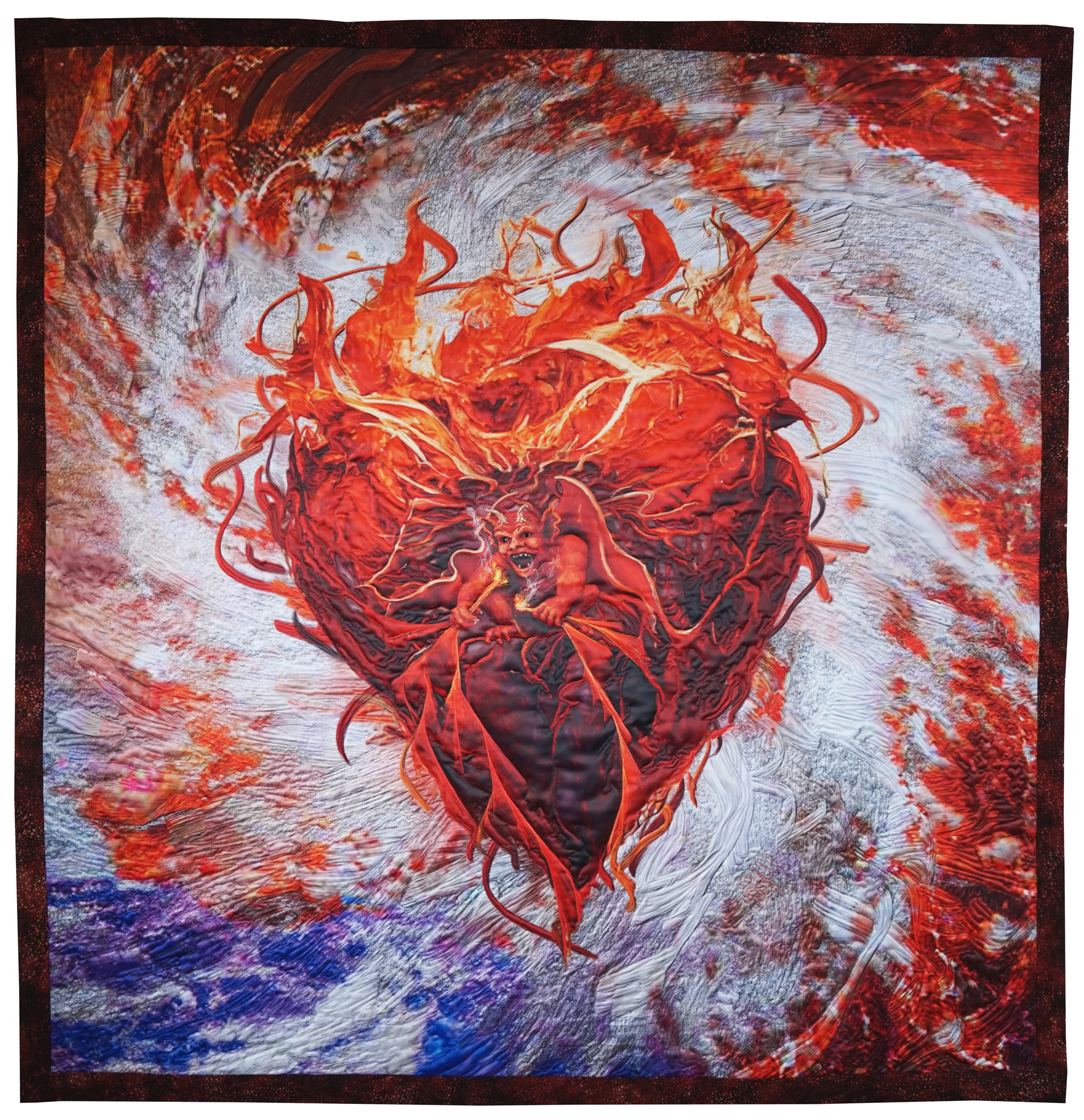This striking square painting, set in a dark brown frame with a speckled rust texture, radiates an intense and almost malevolent energy. The focal point is a heart-shaped structure, stringy and thread-like, its edges seemingly aflame with vivid red and orange hues. The heart’s lower and middle portions are engulfed in a near-black darkness, from which a demonic figure emerges. This creature, an embodiment of fiery red, menacingly displays its horns and extends its hands and feet to grasp strands forming the heart. Its mouth is agape as if it is surging towards the viewer, slightly to the left. The background is a chaotic whirlpool of colors: white brushstrokes create a pinwheel effect from the center, transitioning to fiery reds and oranges, and finally blending with dark blue and white hues in the lower sections. This surreal and dramatic illustration elicits a sense of unease and powerful visual impact.